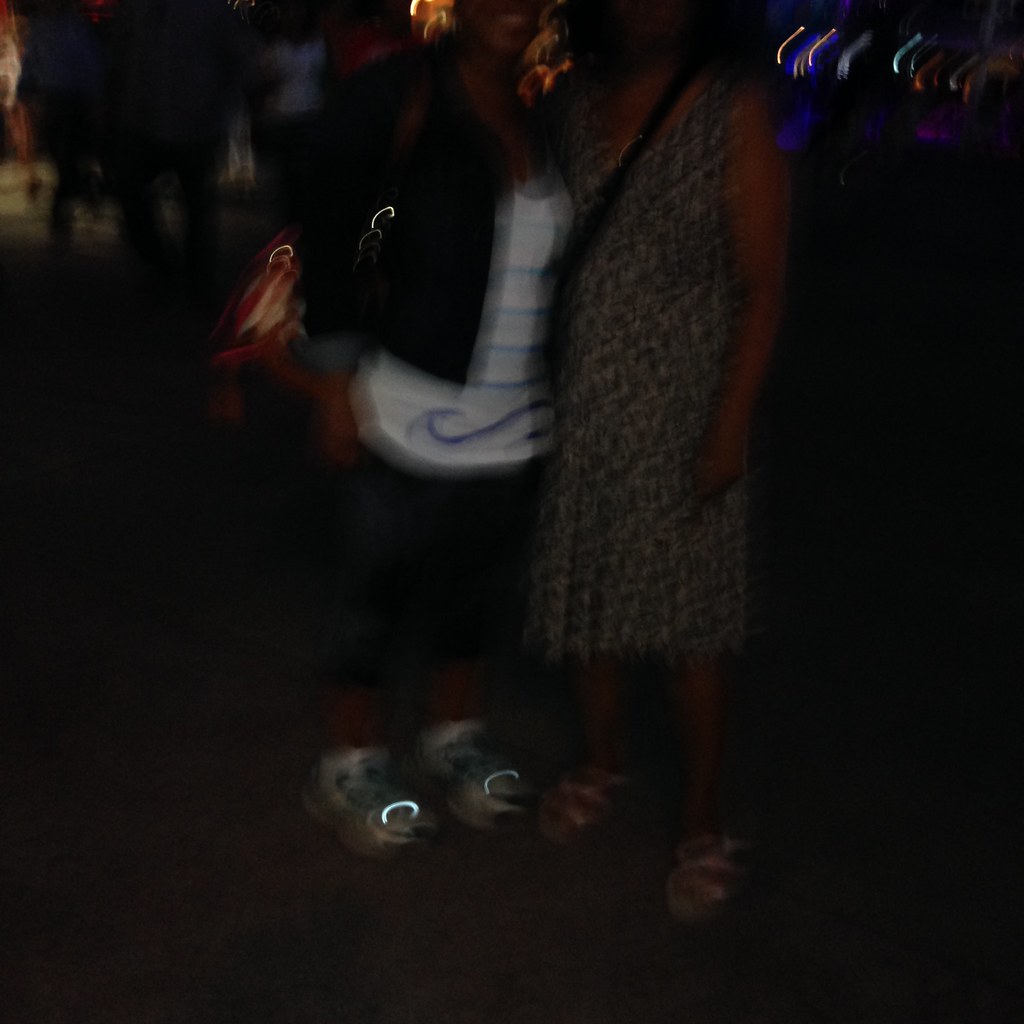The image captures a blurry nighttime scene featuring two women standing close together, facing the camera with their heads cropped off just above their noses. The woman on the left is dressed in a black jacket over a white shirt with blue horizontal stripes and blue jeans or capris. She wears tennis shoes with semi-circular lights on them and holds a reddish handbag with a brown strap over her right shoulder, tassels noticeable on the bag. Her hair slightly comes into view on the right side of her face, and she seems to be holding something indistinct. The woman on the right wears a long, black and white spotted dress, extending to her ankles, and white sandals with mini straps. She has a strap across her torso, likely from a handbag. The background is dark, adorned with streaky lights and spots, and depicts silhouettes of other people and various light streaks, creating a sense of movement. Overall, the image exudes a dynamic and somewhat mysterious atmosphere, enhanced by the motion blur and out-of-focus elements.